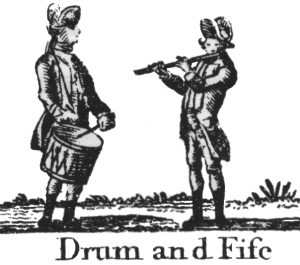This image is a very simple, black-and-white, low-quality drawing titled "Drum and Fife," potentially depicting a scene from the American Revolutionary War or the Civil War era. It features two men in detailed military uniforms, complete with ornate hats or helmets, long-tailed waistcoats, tight pants, and high knee boots or leggings. Both figures are standing on minimal ground cover that appears to be dirt or grass. The man on the left is playing a fife, holding it to his lips and looking down at the instrument. The man on the right, who is slightly taller, carries a single drum tied around his neck, playing it with drumsticks while looking at the fife player. The background is minimal and transparent, emphasizing the two musicians against the sparse outdoor setting without any additional context like buildings or other people. This meticulously hand-drawn illustration suggests the historical importance of military music as part of a fighting regiment's morale and communication.